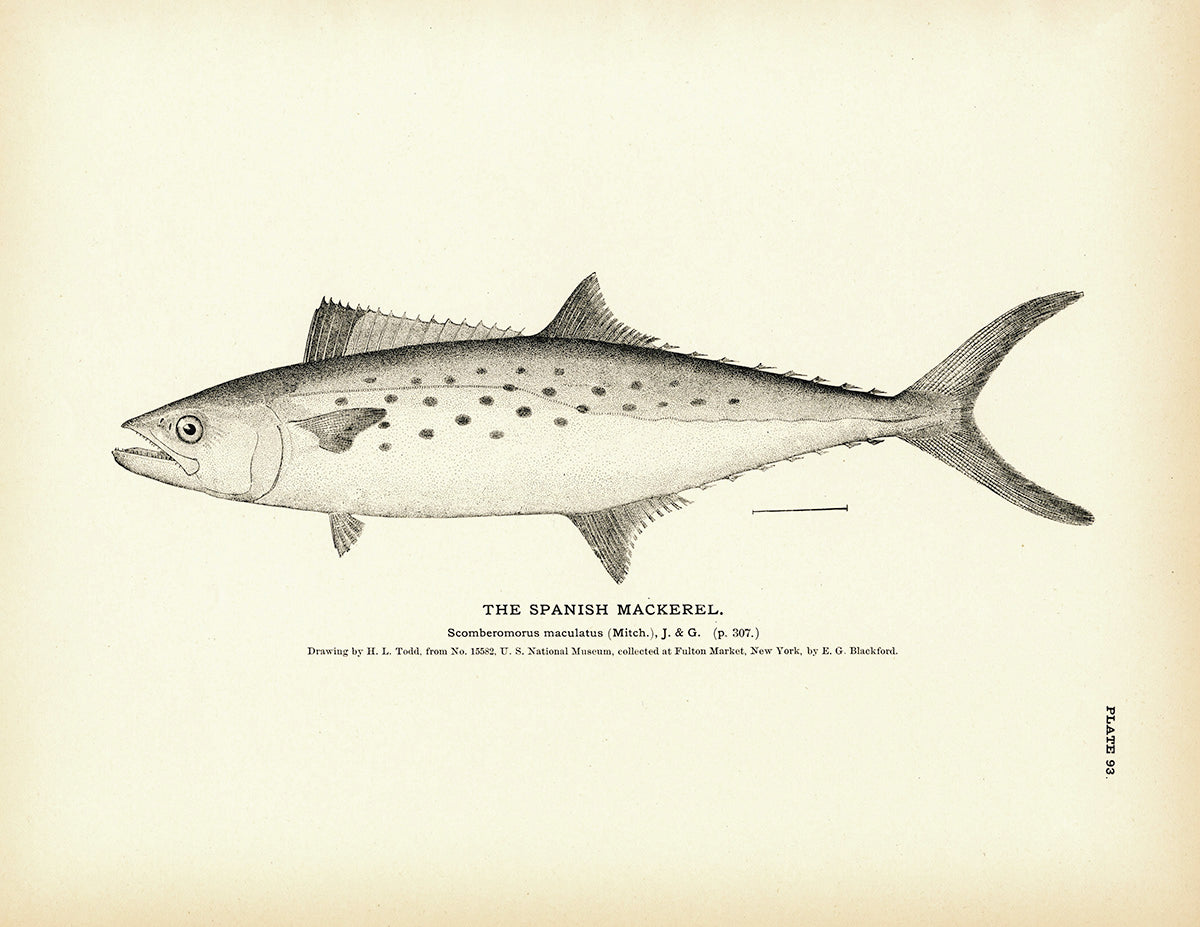This black-and-white pencil drawing by H.L. Todd showcases a highly detailed side view of a Spanish mackerel (Scumberomus maculatus). The textured illustration features intricate crosshatching, particularly on the fins, contributing to a three-dimensional effect. Below the fish, the description reads: "Spanish mackerel, Scumberomus maculatus. Drawing by H.L. Todd from number 15582, U.S. National Museum, collected at Fulton Market, New York by E.G. Blackford." Additional annotations include "Cicumbris maculitis" along with "J-N-G" and "page 307." On the right side, the vertical text "plate 93" is present. The fish is depicted with gaping mouth, prominent eye, five fins, and a tail, against a clear white background.